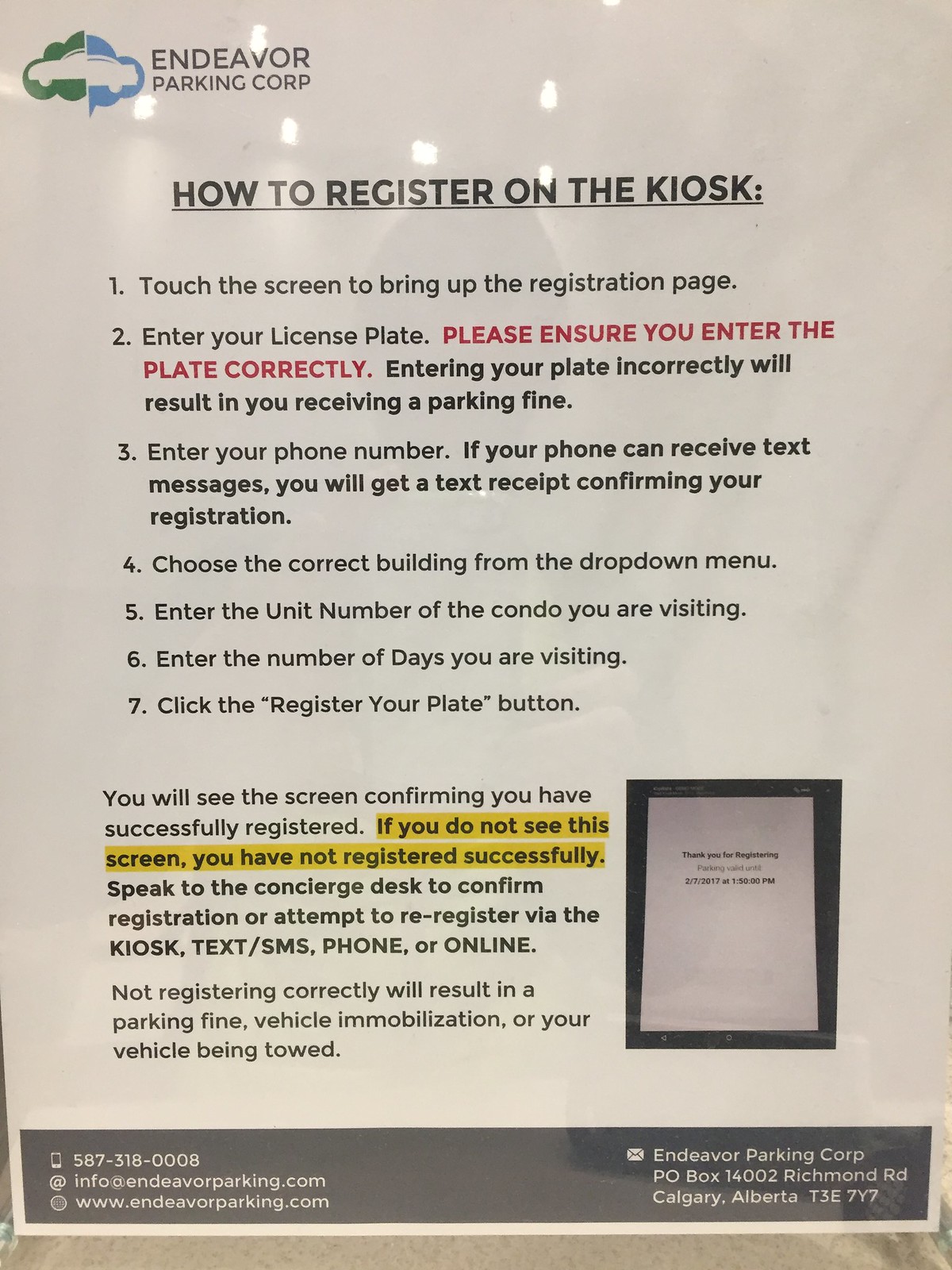The image is of a detailed sign or notice from Endeavor Parking Corporation, providing step-by-step instructions on how to register your vehicle on their kiosk. The document, which appears to be propped up on a surface, begins with the company's logo and the title "How to Register on the Kiosk." The steps outlined are as follows:

1. Touch the screen to bring up the registration page.
2. Enter your license plate. Please ensure you enter the plate correctly, as entering it incorrectly will result in a parking fine.
3. Enter your phone number. If your phone can receive text messages, you will get a text receipt confirming your registration.
4. Choose the correct building from the drop-down menu.
5. Enter the unit number of the condo you are visiting.
6. Enter the number of days you are visiting.
7. Click the "Register Your Plate" button.

The sign emphasizes that you will see a confirmation screen if you have successfully registered. If you do not see this screen, you have not registered successfully and should speak to the concierge desk or attempt to re-register via the kiosk, text or SMS, phone, or online. Failure to register correctly can result in a parking fine, vehicle immobilization, or your vehicle being towed. For further assistance or information, the sign provides contact details including a phone number (587-318-0008) and an email address (info@endeavorparking.com), as well as a website (www.endeavorparking.com). The company's mailing address is P.O. Box 14002, Richmond Road, Calgary, Alberta, T3E7Y7.